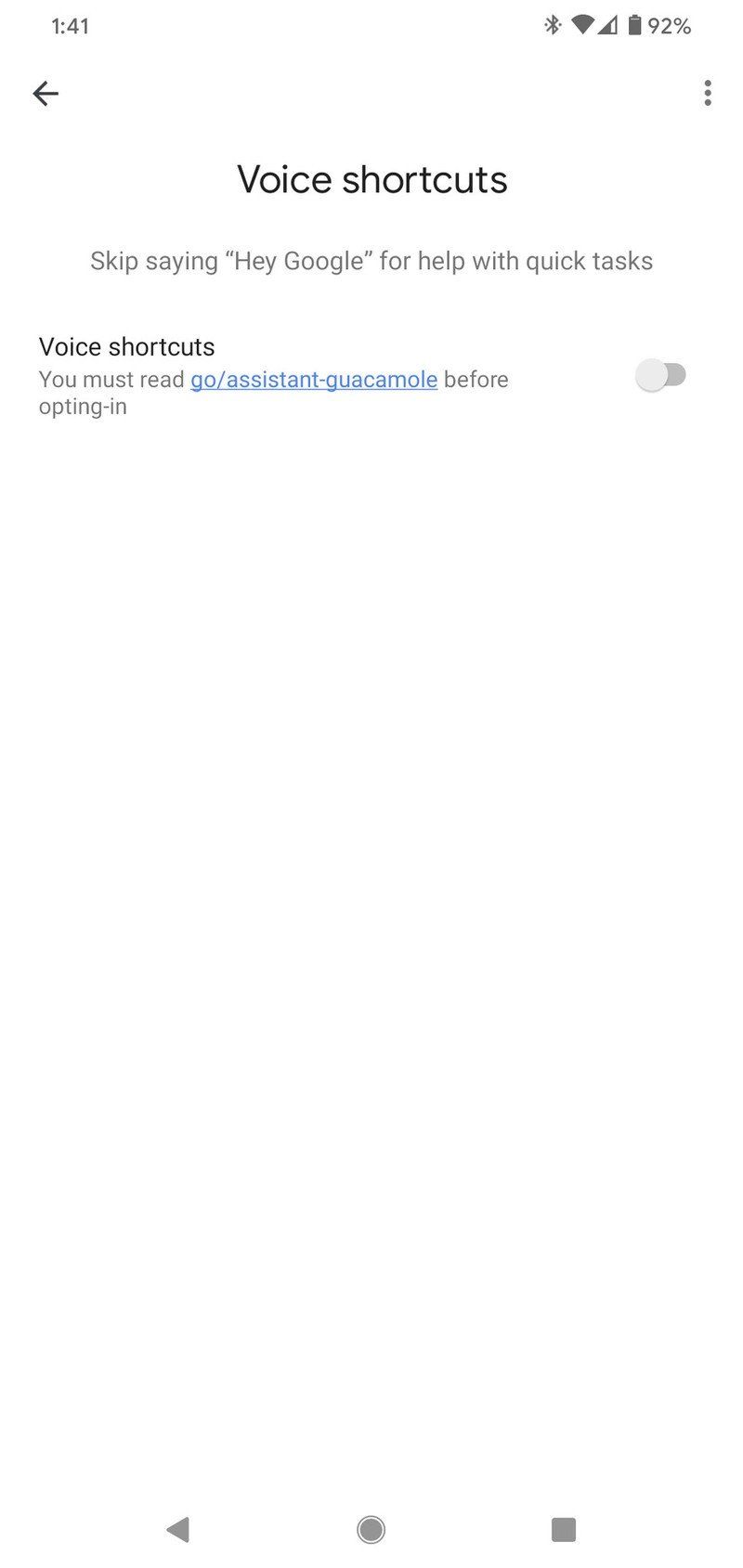The image is a vertical-oriented screenshot from a mobile device with a clear white background and substantial empty space. It lacks any distinctive border. 

At the upper left corner, the time is displayed as 1:41. The upper right corner shows four icons, including Bluetooth, Wi-Fi, and a battery icon indicating a 92% charge. Below these, on the far left, there is a left-facing arrow, and on the far right, there are three vertical dots representing a menu.

Centrally located below these icons is the heading "Voice Shortcuts" in prominent text. Beneath this heading, a smaller gray text states, "Skip saying, Hey Google, for help with quick tasks."

Further down, in the shortcut section, the heading "Voice Shortcuts" reappears. Below it is an important instruction: "You must read," followed by a blue, underlined hyperlink reading "Go/assistant-guacamole" indicating the user needs to navigate to this link before opting in. To the right of this text is a small gray slider, currently switched off.

At the very bottom of the image, floating navigation icons are present: a left-facing gray arrow, a gray circle, and a gray square, each filled in with a matching gray fill.